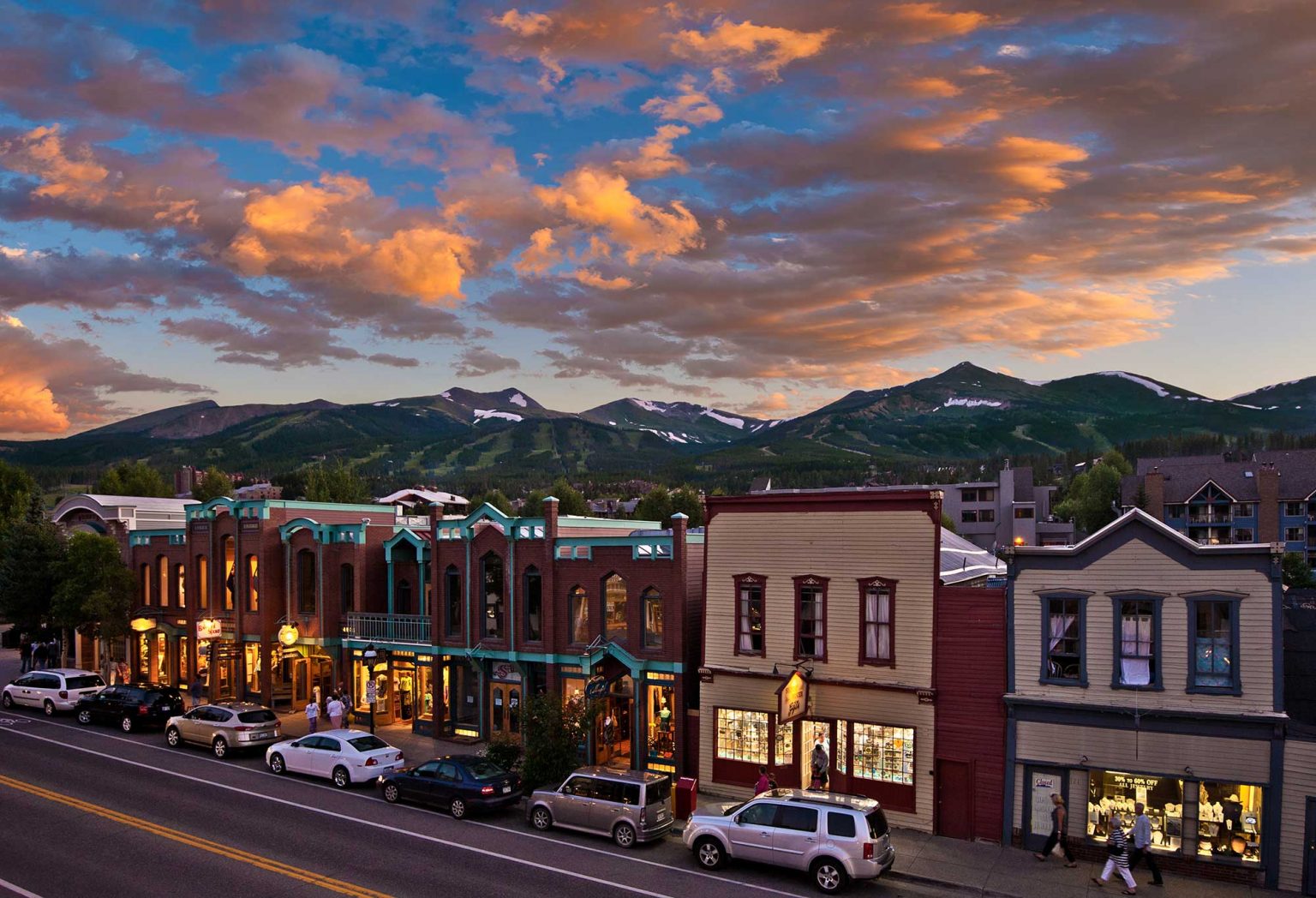This drone-shot photograph captures the essence of a quaint, historic downtown district. Taken from approximately 20 feet above ground at dusk, the image showcases a serene evening scene under a blue sky adorned with white clouds tinged pink and yellow by the setting sun. The picturesque backdrop features rolling green hills and towering mountains with sparse patches of snow, hinting at a temperate climate. 

The main street below, paved with black asphalt and marked by a double yellow line, is flanked by two-story buildings dating back to the early 20th century. These structures display a charming mix of architectural styles and colors: some are constructed from red and white brick, while others are wooden with flat square faces. Shopfronts on the lower levels are warmly lit, indicative of bustling businesses within. Pedestrians stroll along the sidewalks, passing an assortment of vibrant storefronts with varied accents in blue, red, and green. Several cars are parked along the curb, contributing to the lively yet peaceful ambiance of this old-timey, small-town setting.